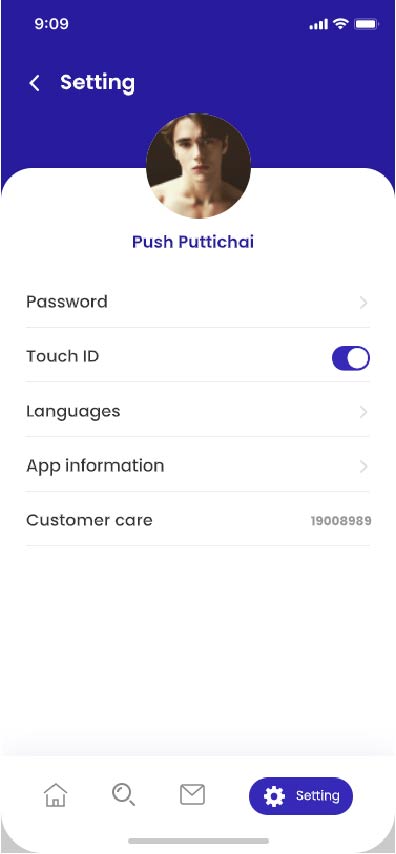This image displays the settings menu on an iPhone. At the very top, a bar shaded in bluish-purple shows the time as 9:09 on the upper left, with fully maxed-out cell and Wi-Fi signals and a full battery icon on the upper right. Directly below the time, there is a white back arrow labeled "Settings."

In the center portion of the bluish-purple area, transitioning into the white section, there is an avatar of a clean-shaven male. Beneath the avatar, the text “Push” is displayed, followed by the name "PUTTICHAI."

Several tabs are listed below the avatar, including:

1. **Password & Touch ID** - This feature is enabled, indicated by a switch toggled to the right.
2. **Languages**
3. **App Information**
4. **Customer Care** - Contact number listed as 1900898989.

At the very bottom of the screen, a navigation bar features four icons: a home icon, a search button, a mail button, and a settings button, which is highlighted in blue and white.